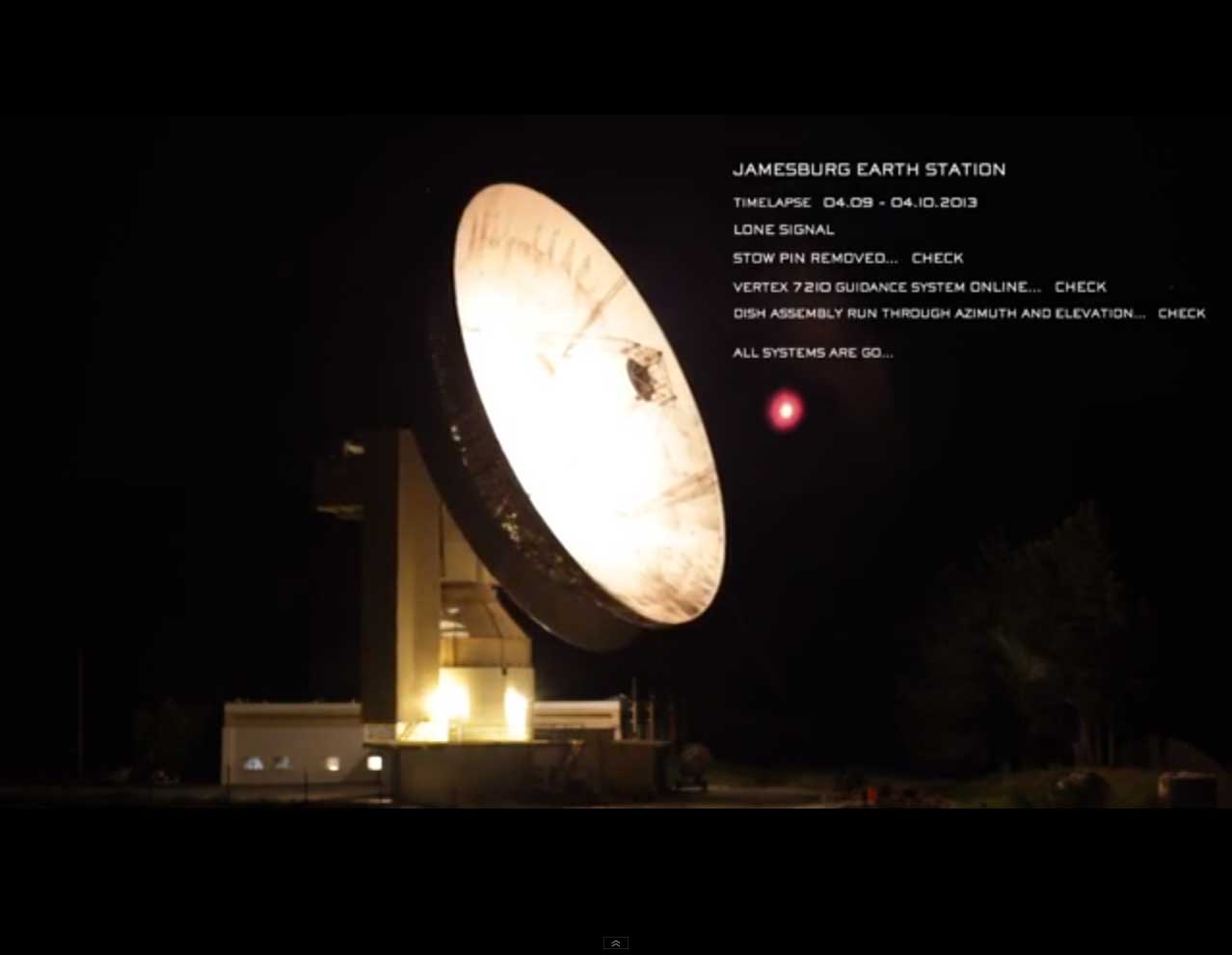The photograph captures the Jamesburg Earth Station at night, framed against a pitch-black sky. Dominating the image is a massive satellite dish, brightly lit from within and angled upwards as if pointing towards the stars. The dish is attached to a large building with multiple sections; the lower sections flank either side of a towering central structure that houses the dish. The building itself is illuminated, with a yellowish glow emanating from lights along its sides and through its windows. Below the structure, the ground is barely visible, hinting at the presence of vehicles parked outside. To the right of the dish, a red flare punctuates the darkness, adding a dramatic touch. Superimposed text reads: "Jamesburg Earth Station, time lapse 04.09 to 04.10.2013. Lone signal, stow pin removed, check. Vertex 7210 guidance system online, check. Dish assembly run through, azimuth and elevation, check. All systems are go."